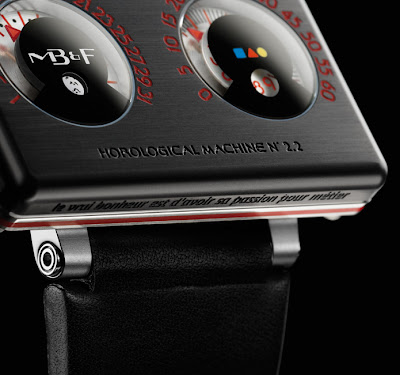This image showcases a unique electronic device, likely a specialized measurement gauge or horological piece, set against a black, shiny, reflective background. The device, labeled "Horological Machine No. 2.2," features a sleek rectangular design with a black rubber or vinyl base and a silver hinge, allowing it to tilt backward slightly. The face of the device is dominated by two distinct dials, each encased in concave clear plastic lenses.

The left dial displays blue, square, red triangle, and yellow circle shapes, while the right dial features the letters M, B, and F. The numeric scales on the dials are unconventional; the left one ranges from 1 to 31 in odd numbers, and the right one progresses in increments of 5 from 0 to 60, all in red text. Both dials include red arrows and needles indicating specific measurements. Additionally, French words appear engraved at the bottom of the device, ending in phrases like "pour," "mince," or "passion pour."

The overall appearance suggests a highly specialized instrument, likely related to horology or precise measurements, standing prominently on a reflective surface that mirrors its base, adding to its sophisticated allure.